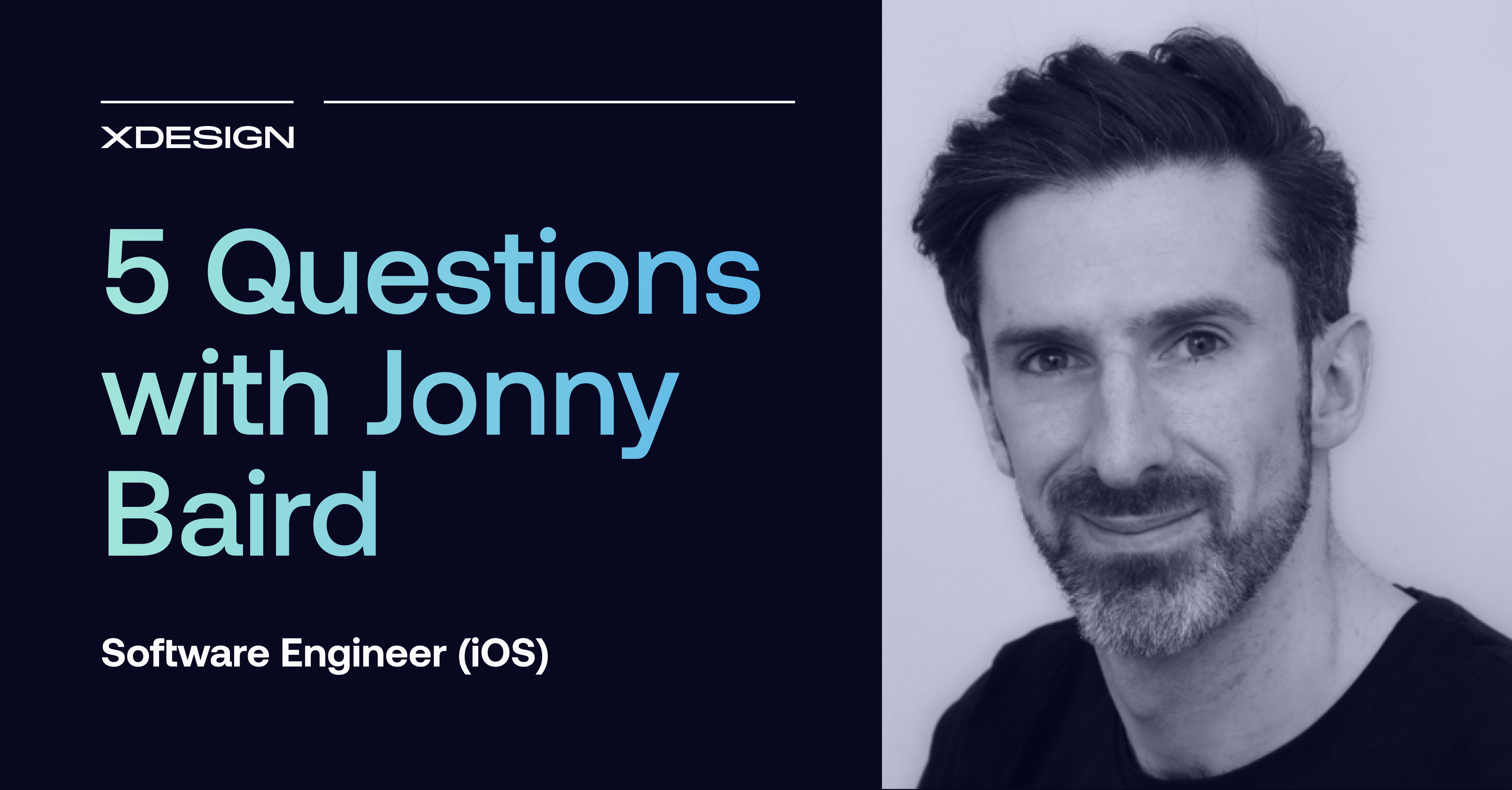The image features a webpage from a website presumably called "XDesign". In the top left corner, there's a thin line followed immediately by the website's name, "XDesign", in white font. Below this, a larger bold text shifts color from turquoise to blue, reading "Five Questions with Jonny Baird". Underneath this title, a smaller white text identifies Jonny Baird as a Software Engineer at iOS. The entire text is presented on a dark blue background. 

Occupying the right side of the image is a photograph of Jonny Baird. He is dressed in a dark shirt, has short dark hair, a mustache, and a salt-and-pepper beard. His image is rendered in a black and white tone with a blue and purple hue, and he looks directly at the camera, filling the whole right half of the screenshot.